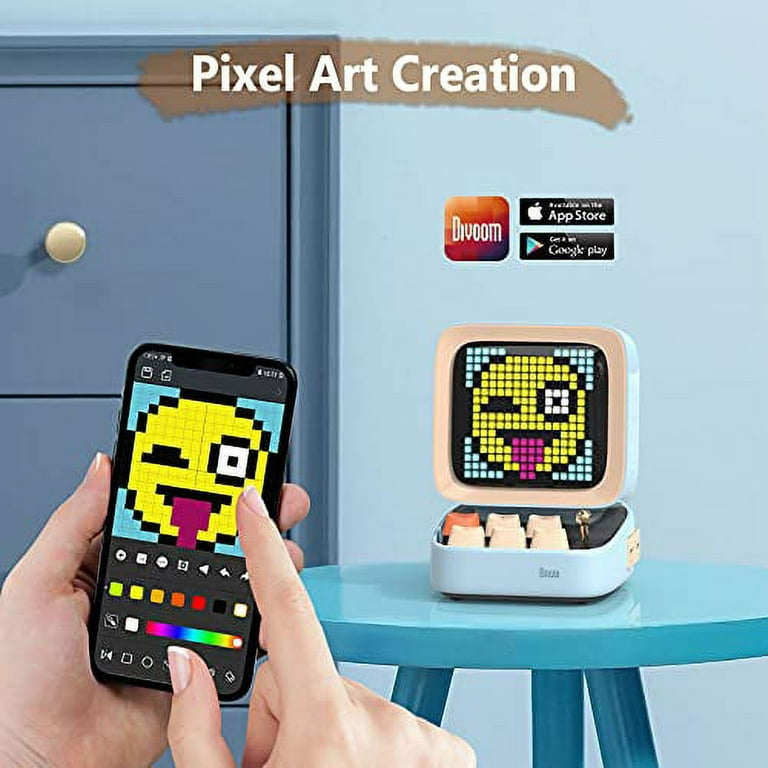In a room with a light blue background, a photograph captures a detailed scene titled "Pixel Art Creation" in a brown, paint-like stroke at the top of the image. The focal point is a pair of well-manicured hands—one of which holds a black smartphone displaying a pixel art app. On the phone screen, there is a customizable page where the user is creating a yellow face emoji with its tongue sticking out. This exact pixel art is also shown on a small retro computer model sitting to the right on a three-legged blue table. The retro device features six buttons, a small screen displaying the same emoji, and text above it reading "DIY OOM" with logos indicating the app's availability on the App Store and Google Play. In the background, there is a built-in blue area with a drawer, and multiple shades of blue color dominate the room's aesthetic.